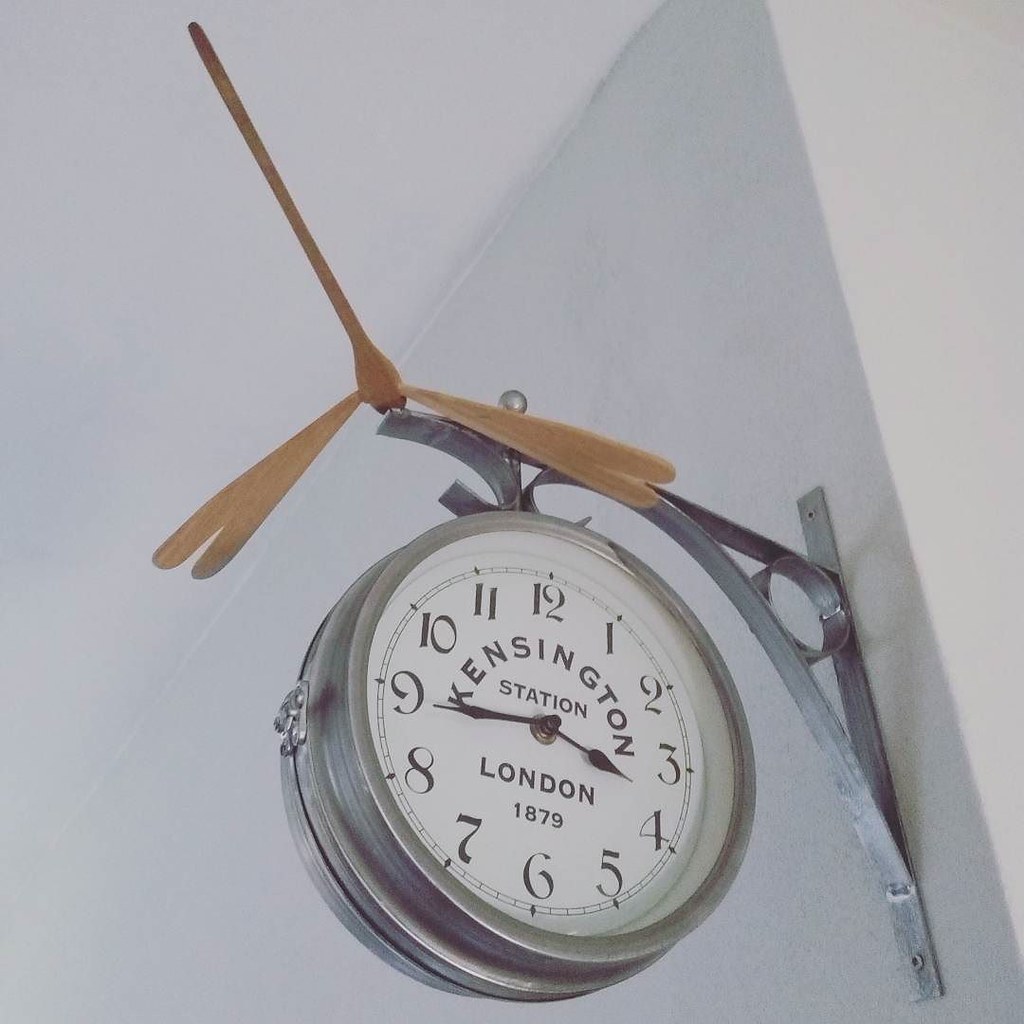The photograph showcases a round clock hanging from a metal bracket mounted on a wall. The clock, marked "Kensington Station, London, 1879," features a white face encircled by a stainless steel rim, with black numbers and hands for hours and minutes. The bracket, a vertical strip of silver metal screwed into the wall, extends outward in a curved, arched arm adorned with an abstract wooden ornament resembling a bird or dragonfly with elongated wings and body. The image is taken from a low angle, revealing part of the white wall and ceiling, with the wall appearing in a light gray hue. The detailed perspective highlights the elegant yet functional design of the clock and its mounting.